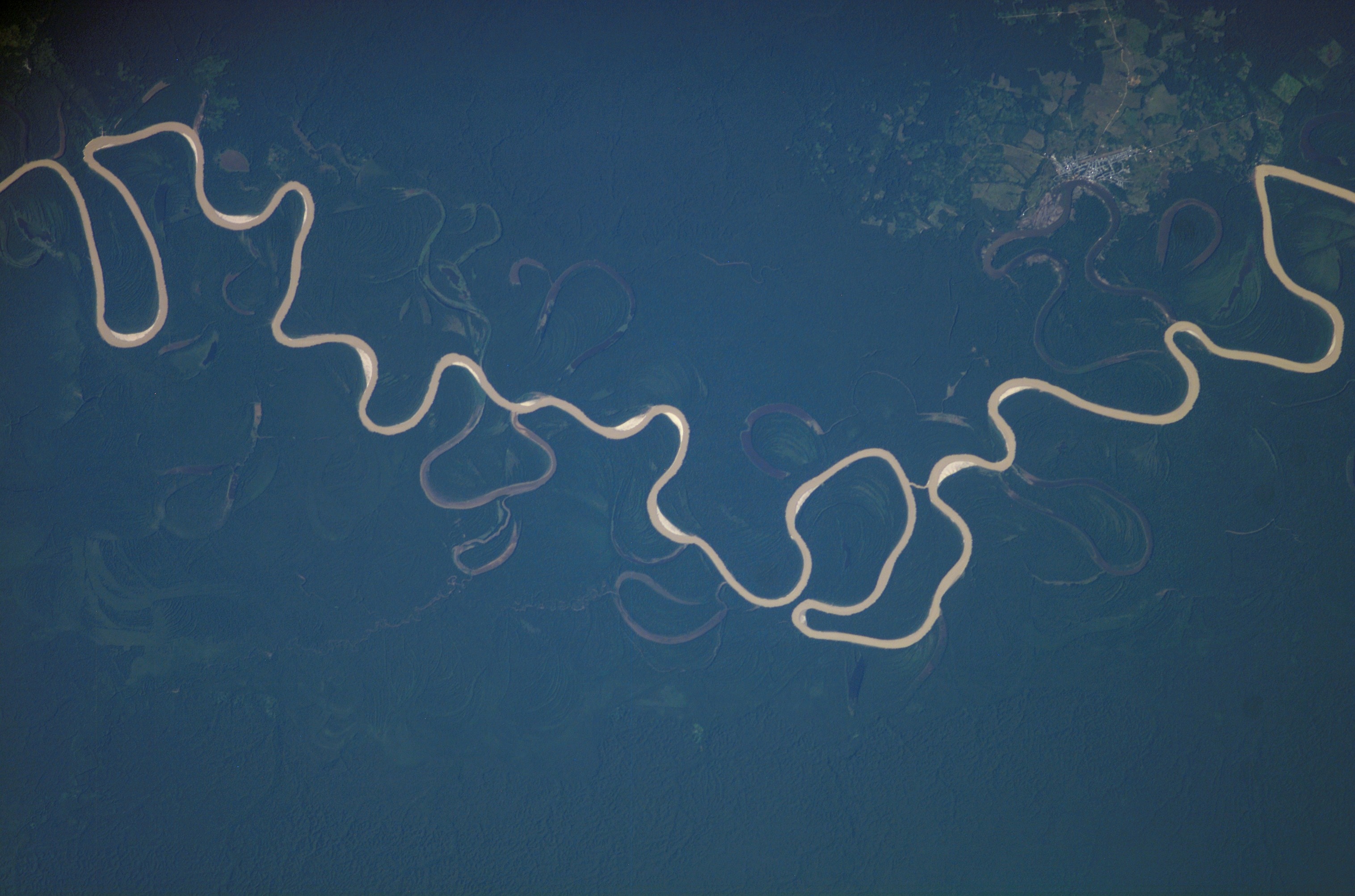This is a horizontally-oriented color photograph featuring an abstract representation of what appears to be the ocean surface. Dominating the image is a foggy, dark bluish-gray expanse that provides a sense of depth and ambiguity. In the top right-hand corner, there are subtle, faded patterns reminiscent of earthly textures seen in satellite imagery, suggesting either landforms beneath the water or cloud formations influencing the visual texture. A delicate, squiggly line of light brown color snakes its way from the top left corner down towards the top right, resembling a thin, viscous substance, possibly a stain or natural occurrence on the water's surface. This irregular line sweeps across the image like a randomly laid string, adding a dynamic element to the serene, muted backdrop.